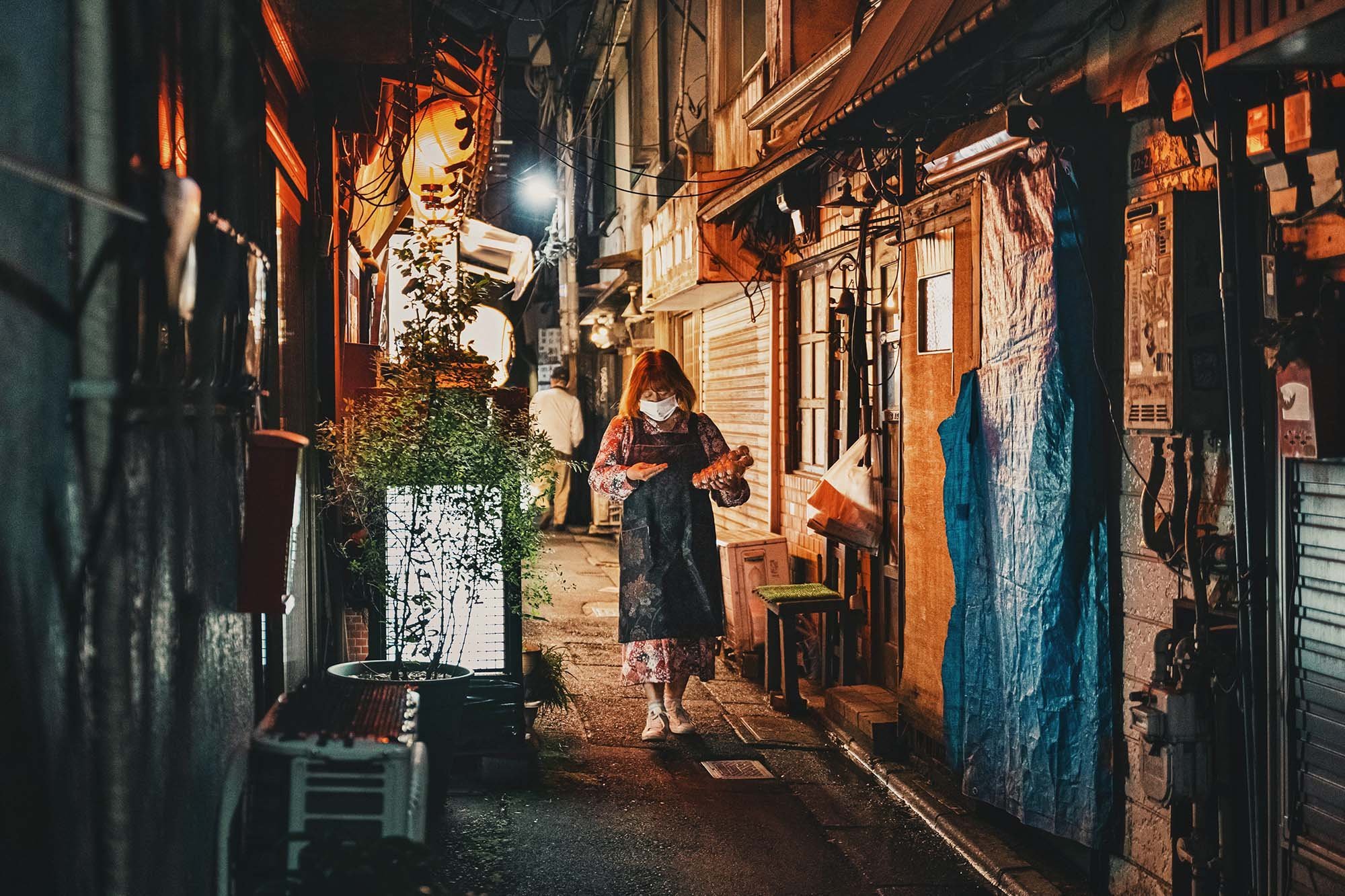The image captures a nighttime scene in a narrow alleyway, likely in Japan, illuminated by numerous street lamps that create a vibrant reflection along the closed shopfronts and stalls. The focal point is a woman wearing a white mask and a flower-patterned dress with a matching blue apron also adorned with flowers. In her left hand, she carries what appears to be eggs, while her right hand holds either a phone or money. The right side of the alley is lined with closed doors and a section covered by a blue tarp. On the left, there is a potted plant and a bench, with another person in the background wearing a white jacket and brown pants. Additional details include a power box affixed to the wall and various items creating a contrasting blend of colors and textures in the dim light.